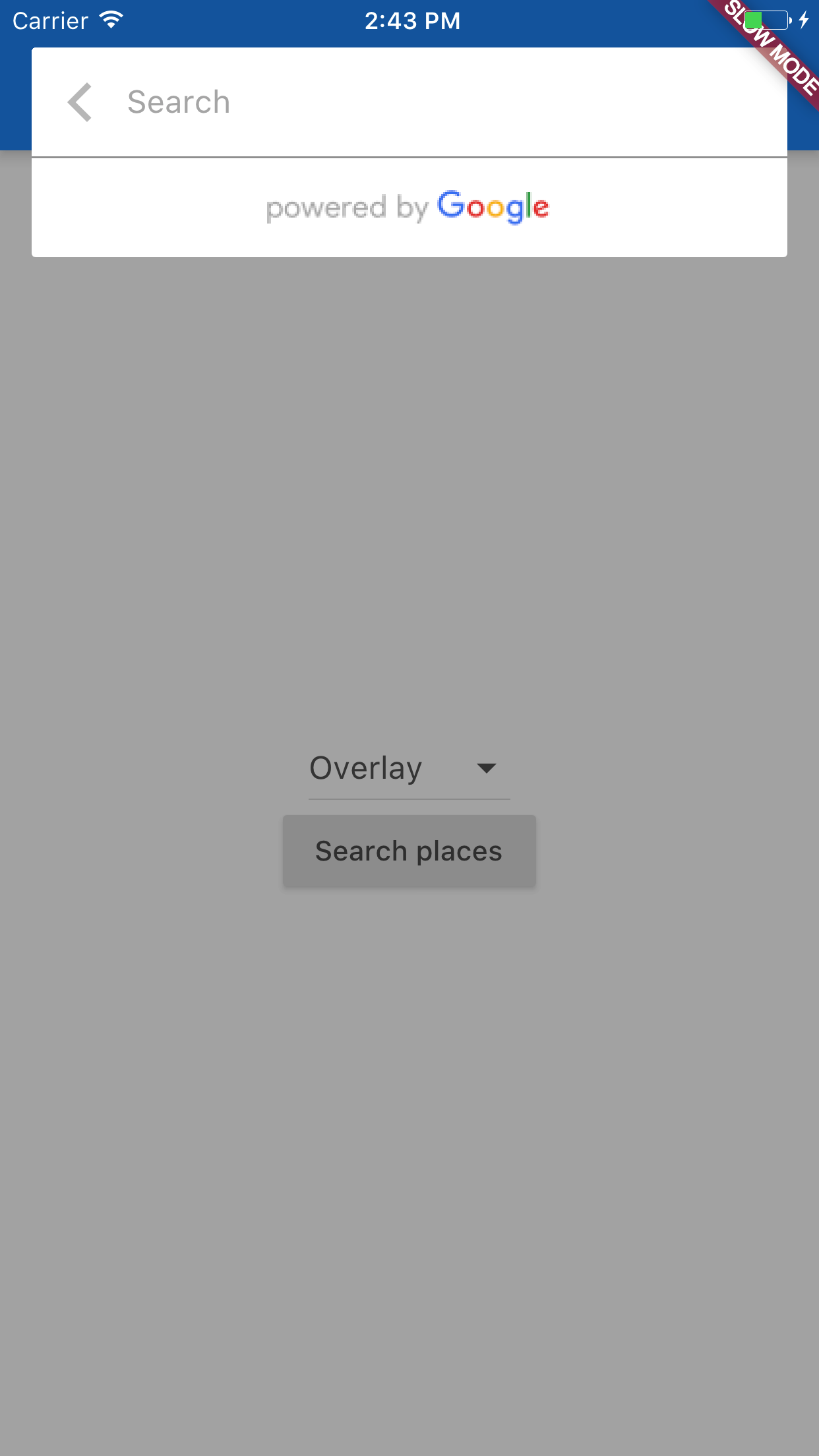This is a detailed description of a color photograph showing a screenshot from a cell phone. The image is rectangular with the longer side oriented vertically. The top portion of the screenshot features a narrow light blue bar, under which the majority of the screen displays a light gray background. 

At the very top of the screenshot, the phone's carrier information and signal strength are visible on the left. In the center, the time is displayed as 2:43 p.m., and on the upper right, there is a battery icon indicating roughly one-third charge with a lightning symbol, signifying that the phone is currently being charged.

Below this status bar, a horizontal white-filled triangle appears at the center, accompanied by the text "Powered by Google." Next to it, there is a search icon with an arrow pointing to the left. 

The central portion of the image prominently features black text that reads "Search," aligned with a downward-pointing arrow. Further below, there is a horizontally-inscribed triangle filled with a slightly darker shade of gray compared to the background. Inside this triangle, in black letters, the text "Search places" is displayed.